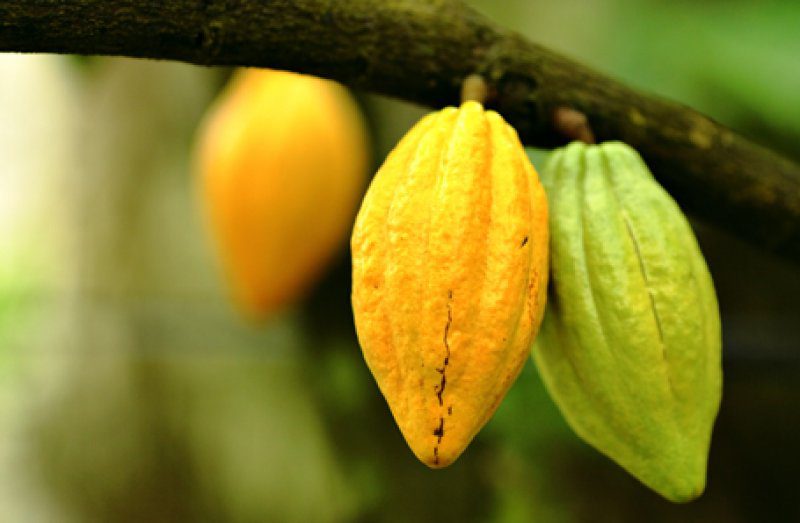The image is a close-up photograph of a tree branch with two distinct fruits prominently displayed in the center. The branch, dark brown in color, extends from the top left corner to about midway down the right side of the image. The central focus is on one bright yellow fruit, suggesting ripeness, and a second pale green fruit, indicating it is not yet ripe. Both fruits are elongated and almond-shaped with notable ridges running from top to bottom. The yellow fruit seems slightly shriveled, likely still hard to the touch, and features some black streaks. In the blurred background, composed of various shades of green and brown, another yellow fruit is faintly visible, blending into the indistinct foliage. The overall composition emphasizes the detailed texture and color of the foreground fruits against an abstract, out-of-focus backdrop.